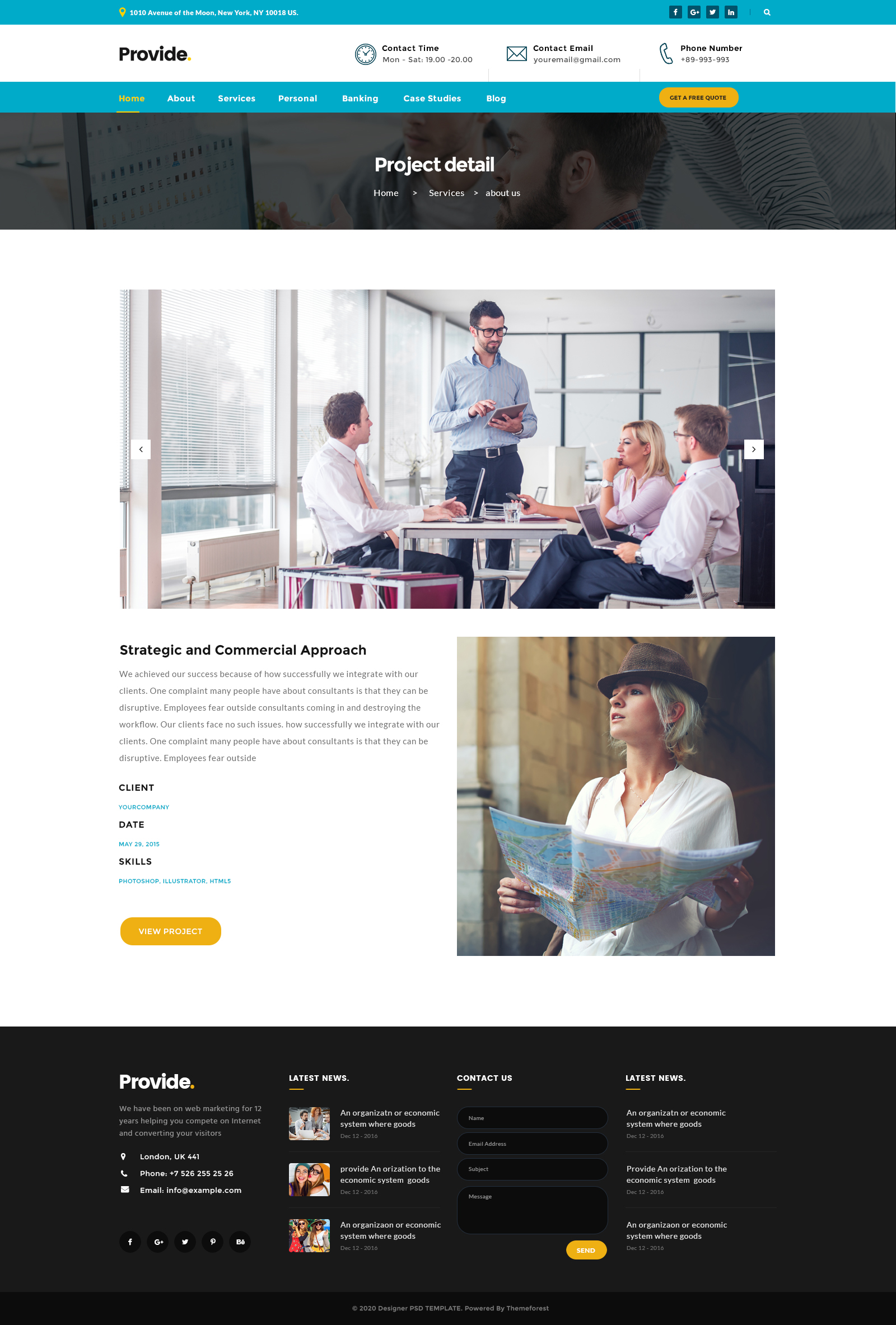The image depicts a business's web page.

At the top left, there's a dark blue bezel displaying a gold pin icon, reminiscent of Google's location pins, with the following text: "Tent and White, 1010 Avenue of the Moon, New York, New York, 10018 US."

Adjacent to this, the company name "PROVIDE" is prominently displayed in bold black text within a large dark gray rectangle. 

On the right-hand side, there's a logo of a clock with the bold text "Contact Time" next to it. Beneath this, in gray text, the business hours are indicated: "Monday through Saturday 1900 to 2000," formatted in military time. 

Below this, an envelope icon is shown with the label "Contact Email," followed by "your.email@gmail.com."

Further to the right, a phone icon is labeled "Phone Number" with the placeholder "+89-993-993," signaling a fake contact number.

In the image, there is also a board meeting in progress. A man wearing a blue dress shirt and blue dress pants, with spectacles and short hair, is leaning over a tablet. At the table, two individuals are sitting to his right—a female with dirty blonde hair in a pink dress shirt, and a male in a white dress shirt with blue pants and a red tie. Both are engaged in the discussion, reacting to the man in blue and another individual on their left side, who is wearing a white dress shirt, a pink tie, and blue pants, and has short hair. 

The office setting is notable for its abundant windows, some with partially closed blinds on the left side and fully closed blinds at the back.